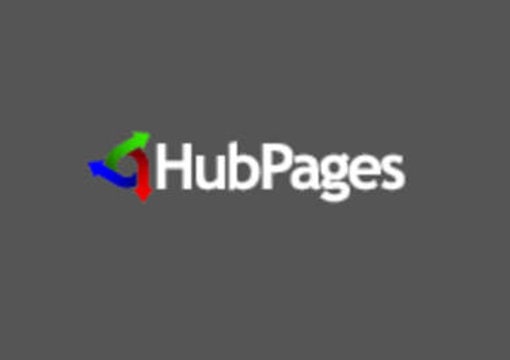The image features a medium to dark gray box centered in the frame. Inside this box, the word "HubPages" is displayed prominently in large, simple white font. The "H" in "Hub" and the "P" in "Pages" are both capitalized, with no space between the two words, making it read seamlessly as "HubPages."

To the left of the text, there are three arrows in different colors. The green arrow curves upwards to the right. Positioned beneath it is a red arrow, which overlaps slightly with the green one. Finally, a blue arrow curves upwards and to the left, partially tucked under the red arrow.

Overall, the design is clean and straightforward, emphasizing the text "HubPages" and its accompanying colorful arrows on a solid gray background.